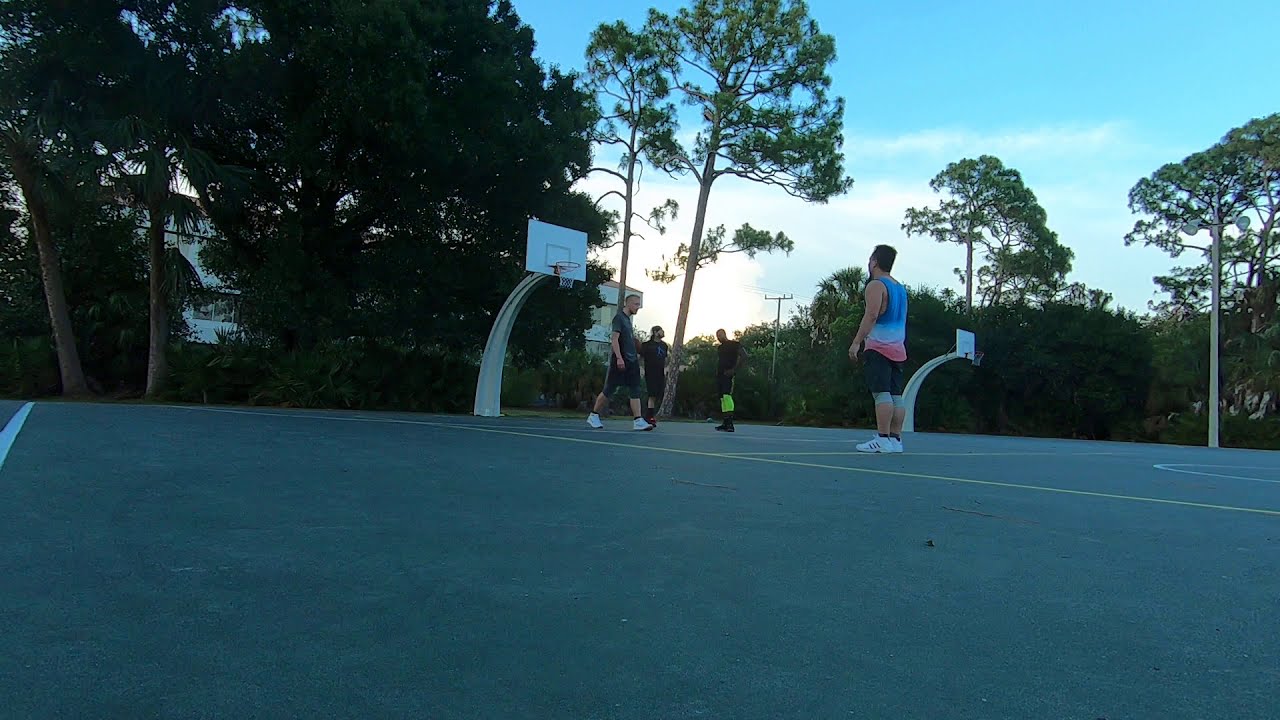The outdoor basketball court features a hard green surface with white boundary lines and yellow markers for different play areas. A unique curved cement pole supports a solid white backboard, which is detailed with a faint red square and an orange rim fitted with a white net. Above, the sky is a vivid blue scattered with white clouds, while the perimeter of the court is framed by trees with brown trunks and green leaves. On the court, four friends are captured in action: the person closest to the camera sports a blue, purple, and pink tank top with blue jeans rolled into shorts; to the right, another friend wears a blue, white, and red tank top paired with dark shorts and white Adidas shoes. Walking towards them is a person in white shoes, dark shorts, and a shirt, while further back, a guy in a black t-shirt, dark pants with a green detail, and another in a backward black hat, black shirt, black shorts, and black shoes, possibly with tall black socks, are engaged in the game. The image appears to be taken from a low angle, as if the camera was placed on the pavement.